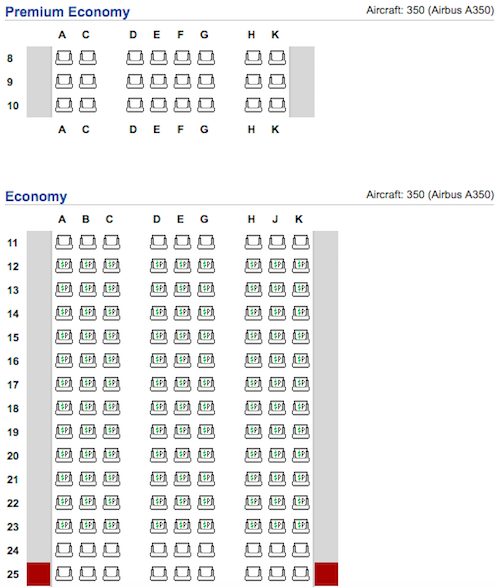The screenshot depicts a detailed seating chart for an Airbus A350 aircraft, highlighting both the Premium Economy and Economy sections. 

In the Premium Economy section, indicated by blue text, the chart lists seat arrangements across columns labeled A, C, D, E, F, G, H, and K. Rows are numbered 8 through 10 on the left side. The seating appears uniform, represented by similar white symbols, likely indicating the placement of seats. 

On the top right of this section, the aircraft model is identified as “Aircraft 350, Airbus A350.”

Below this section, the Economy class is also marked in blue text and repeats the aircraft model designation. The seating chart for Economy includes columns labeled A, B, C, D, E, G, H, J, and K, with rows numbered 11 through 25 on the left. Similar to Premium Economy, seats are uniformly marked with white symbols.

This detailed seating chart provides a clear layout of seat placements for passengers in both Premium Economy and Economy sections of the Airbus A350.